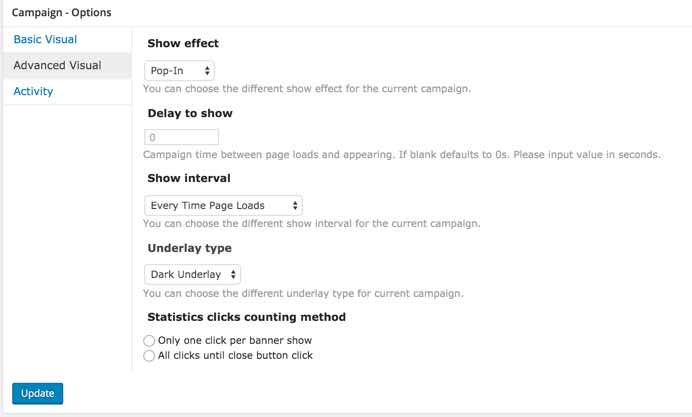Here is a detailed and cleaned-up caption for the image:

---

The image displays a pull-up menu from a campaign site, presenting various configuration options. On the left side of the menu, options are listed in blue text, allowing the user to select between "Basic Visual," "Advanced Visual," or "Activity." The "Advanced Visual" tab is currently selected.

Within the "Advanced Visual" settings, several customization options are available. First, there is a feature to configure the "Show Effect," with "Pop-in" being the selected effect for the current campaign. Below that, there is an input field labeled "Delay to Show," which is currently set to zero seconds. This controls the time delay before the show effect takes place upon page load, with instructions specifying to input the value in seconds.

Next, there is a selection for the "Show Interval," with the option set to "Every time page loads." A description below specifies that users can choose different show intervals for the current campaign. The "Underlay Type" is configured as a "Dark Overlay," with an accompanying description indicating that this setting determines the background appearance behind the visuals.

Lastly, the menu includes an option for the "Statistics Clicks Counting Method." Users can choose between "Only one click per banner show" or "All clicks until close button click." 

At the bottom left of the menu, there is a button labeled "Update," displayed in red font against a blue background, which provides the functionality to save any changes made to the settings.

---

This caption provides a clear and comprehensive description of the menu options and their current configurations.